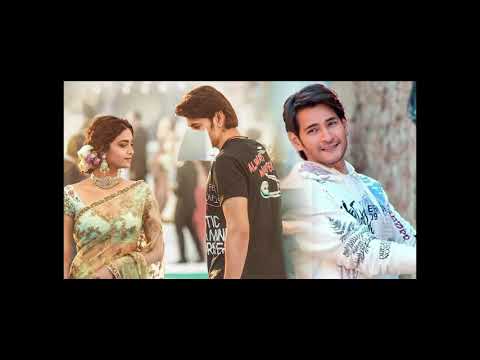The image is a composite of two photographs blended together. On the left side, it features a young couple with the woman dressed in formal Hindu attire. She is wearing a silky green dress decorated with intricate beadwork and floral patterns, complemented by a see-through sash that drapes gracefully over her arms. Her hair is pulled back into a low bun adorned with a cluster of flowers, and she wears drapey earrings and a jeweled necklace. She is facing the man beside her, her gaze directed towards him. The man, who appears slightly out of place next to her, is dressed casually in a black graphic t-shirt. His straight brown hair is short and swept over to one side, and he seems to be looking down, with his face partially obscured or blurred. In the background, there is a crowd of people, though they are indistinct and blurred. The right side of the image features a portrait of a man with darker brown hair, sitting and facing the camera with a friendly smile. He wears a white long-sleeved shirt with light blue graphics, and the two sections of the image are seamlessly blended, creating an interesting juxtaposition of formal and casual elements.